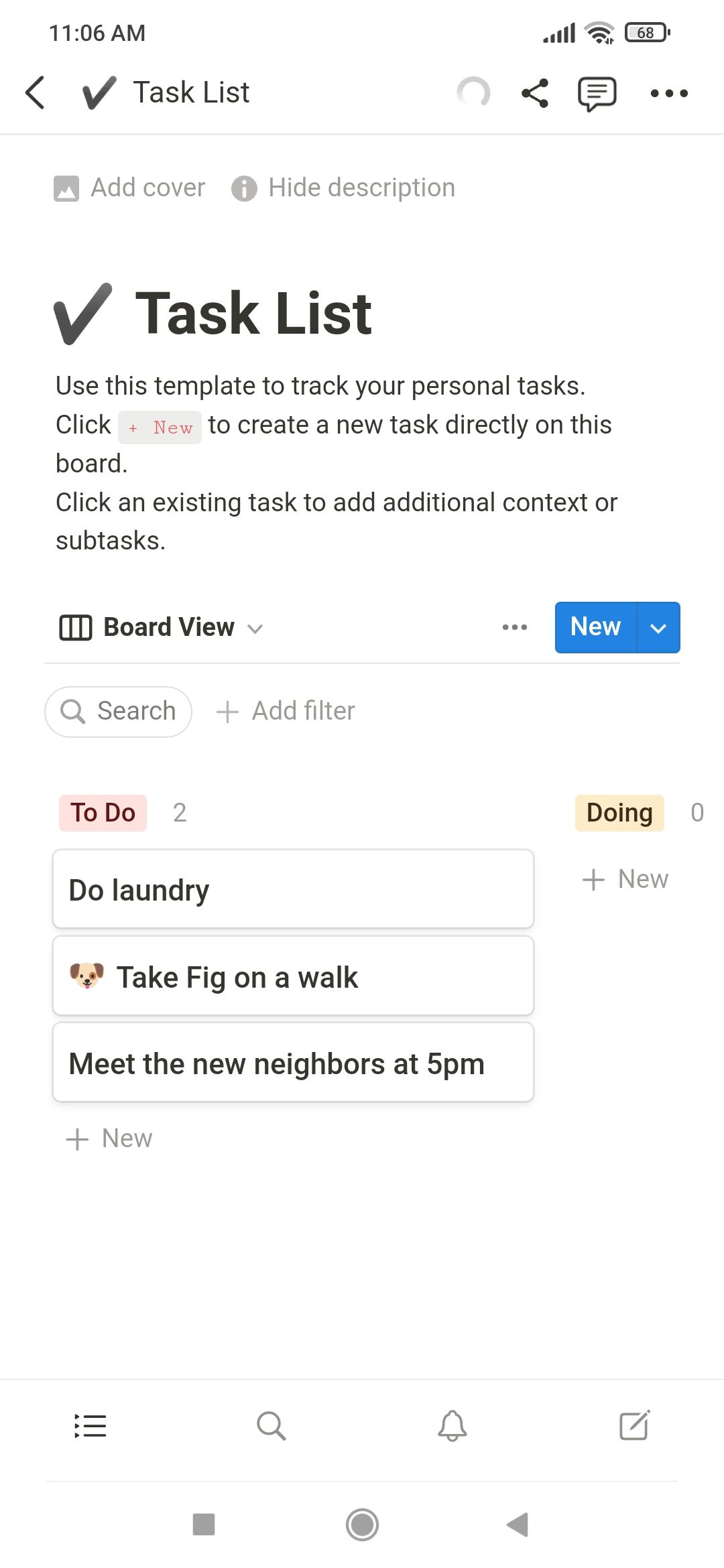The image is a cell phone screenshot, displaying a task management app interface. At the top left corner, the system time is visible, and to the top right are the battery, reception, and Wi-Fi icons. Directly below, there is a navigation bar featuring a left-pointing gray arrow, a bold black checkmark, and the title "Task List." On the same line to the right, icons for sharing text and an ellipsis menu are present.

The next line features the options "Add Cover" and "Hide Description," each accompanied by an icon, displayed in gray. A couple of lines down, there's another bold black checkmark on the left next to the text "Task List" in bold black. This is followed by a description in gray: "Use this template to track your personal tasks. Use the gray 'New' button to create a new task directly on this board. Click an existing task to add additional context or sub-tasks."

Further down, there is a board icon followed by "Board View" in bold black with a gray down-pointing arrow. On the right, there's another ellipsis menu. Below this is a blue drop-down box labeled "New" with white text. Underneath that, there is a search oval and to its right, a plus sign for adding filters.

Towards the bottom left, a section labeled "To Do" is displayed in bold black on a light pink background with a gray number "2" to its right. On the right side, "Doing" is displayed in bold black with a yellow background and a gray "0" next to it. Below these sections, there are task items listed in gray outlined rectangles: 
- Do laundry
- Take Fig on a walk
- Meet the new neighbors at 5 p.m.

These tasks are stacked vertically, providing a clear view of the to-do list.